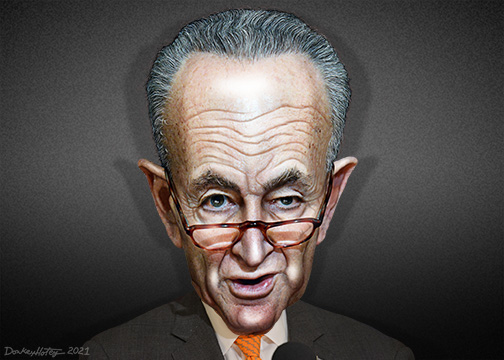A detailed portrait of a comic book character is depicted in this image. Dominating the frame is a man whose exaggerated head takes up a significant portion of the picture, extending from near the top of the image to halfway down. His hair is a mix of gray and black streaks, contributing to his unique appearance. He has elongated ears, reminiscent of an elf's. His eyes add an interesting asymmetry: the left eye is wide open, while the right eye looks as though it is about to close. The man is dressed in a brown suit paired with a cream-colored shirt and an orange tie, further enhancing his distinct persona. Additionally, he sports glasses, giving him an air of intellect and sophistication. The background is very dark, ensuring that all attention remains on the character's whimsical and intriguing features. Despite his unusual appearance, his expression conveys calm and contentment.